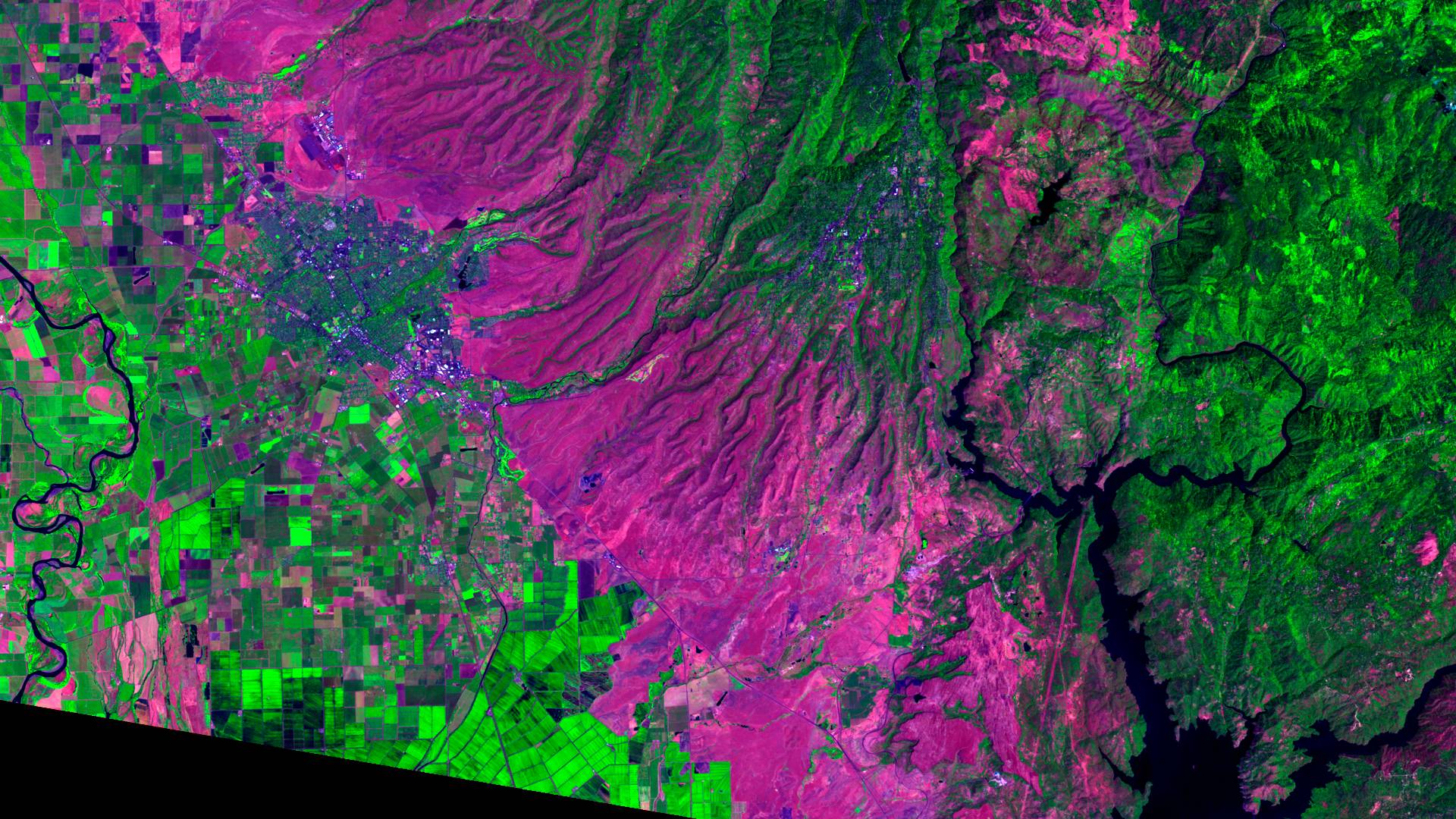This image, which appears to be a color-coded satellite photograph or an abstract painting, depicts a vibrant and detailed landscape. To the left, it is dominated by numerous rectangular and square shapes in various shades of green, indicating clustered buildings or arable land. Interspersed amongst these greens are touches of purple and dark blue, suggesting a transition in terrain or crop types. The central and upper left portions feature smaller squares and rectangles that shift from green to deep purple and dark blue. 

A prominent feature, a very dark almost black snaking shape that resembles a river, runs from the far left to the center. This river-like formation carves through the landscape, with clustered buildings right up to its edge, descending from a vividly purple base of a mountain. This mountain spans the right and center of the image, with colors transitioning from deep purple at the bottom to progressively lighter greens as it extends upward and to the right. The upper right corner of the image also contains a noticeable splotch of purple. The overall composition is a rich mosaic of colors and shapes, beautifully blending to illustrate mountainous terrain, agricultural plots, and possibly riverine systems.